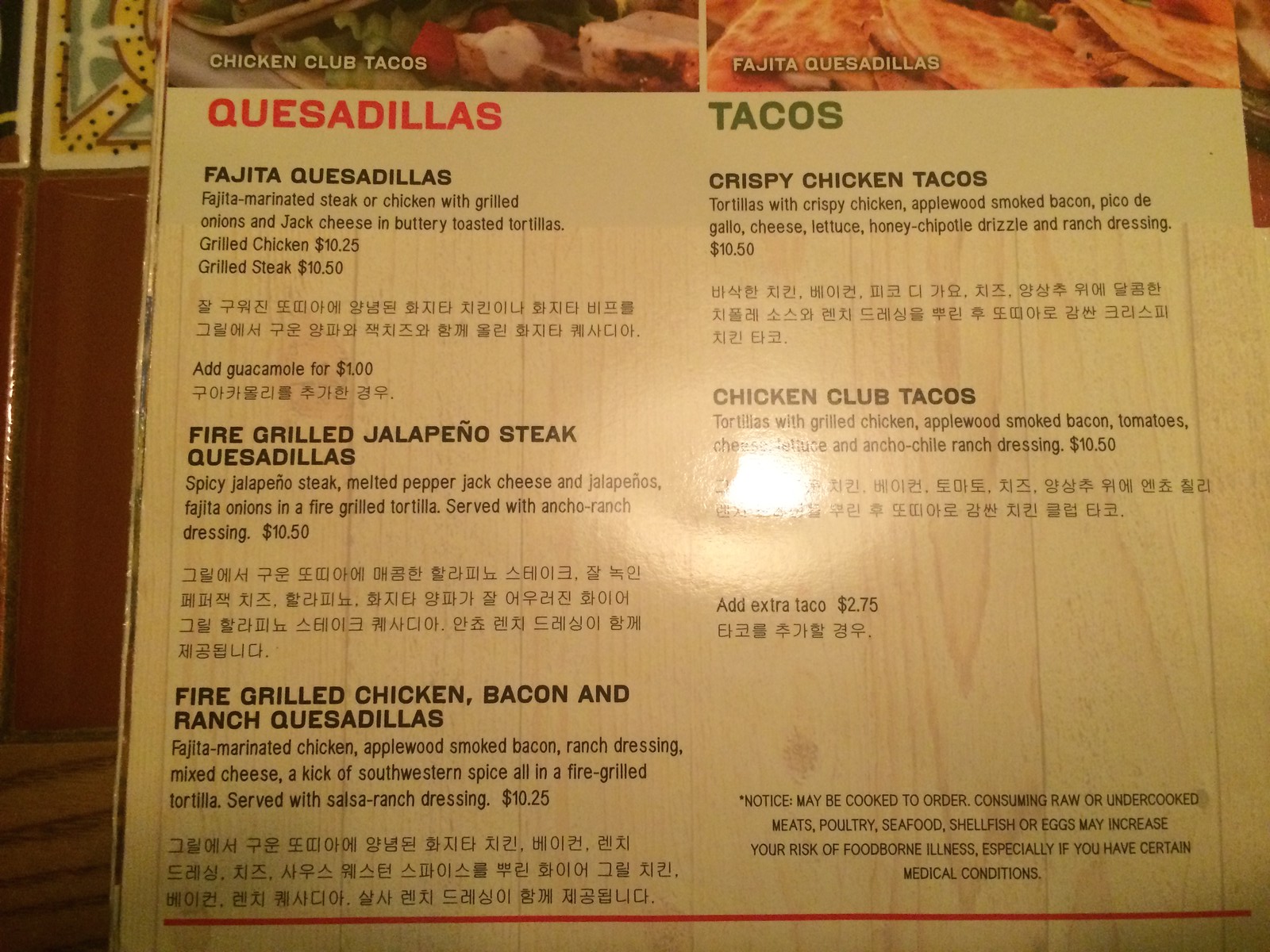This detailed and descriptive caption provides a clear image of the menu:

---

The menu, likely from a Mexican restaurant, features an off-white, slightly yellowish hue. The left section of the menu offers an array of quesadillas, including Fajita Quesadillas, Fire-Grilled Jalapeño Steak Quesadillas, and Fire-Grilled Chicken, Bacon, and Ranch Quesadillas. The prices are listed as $10.25 for both the Grilled Chicken and the Fire-Grilled Chicken, Bacon, and Ranch Quesadillas, while the Fire-Grilled Jalapeño Steak Quesadillas are priced at $10.50. An additional note mentions that guacamole can be added for $1.

On the right side, the menu lists taco options such as Crispy Chicken Tacos and Chicken Club Tacos. Crispy Chicken Tacos are available for $10.50. Customers can opt for an extra taco for $2.75. An important food safety notice is included, highlighting the risks associated with consuming raw or undercooked meats, poultry, seafood, shellfish, or eggs, especially for those with certain medical conditions.

Furthermore, there are small images accompanying the text, showcasing Chicken Club Tacos and a Fajita Quesadilla. 

One intriguing element of the menu is the seemingly out-of-place reference to "Japanese fried" at two different spots, suggesting a possible mix-up or unusual fusion dish.

---

This caption provides a vivid and organized depiction of the menu contents and highlights, enhancing the reader's understanding of its offerings.